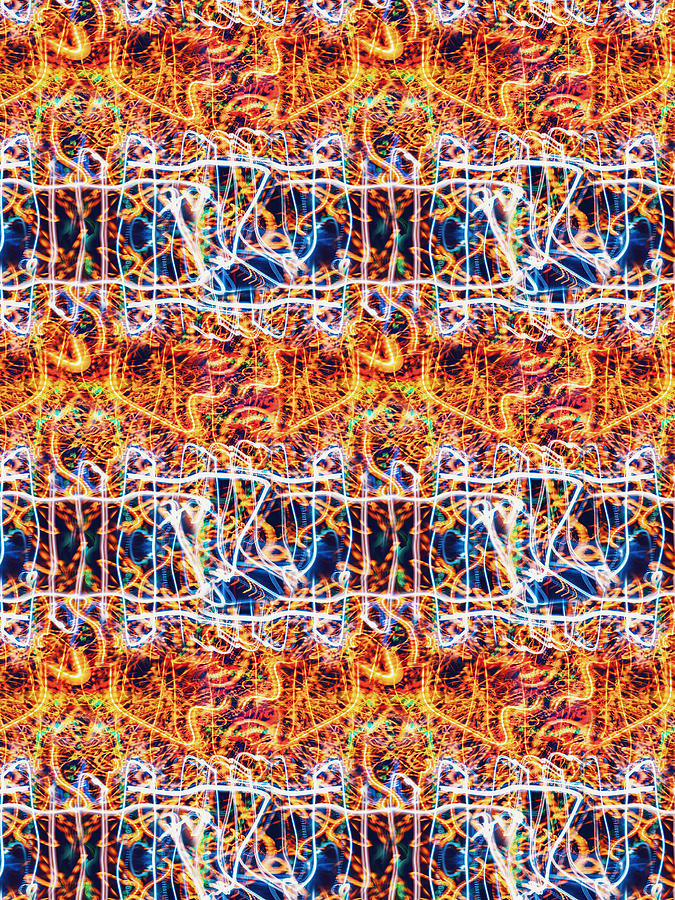This image appears to be a highly intricate and abstract piece of art characterized by interwoven, brightly colored zigzag patterns that resemble neon lights or intricate tapestry. The composition features repeated sequences of colors, primarily gold, blue, and shades of neon green, orange, and white, forming an elaborate, semi-chaotic visual effect. The top section of the image showcases a gold background with zigzag patterns that look like bent pipe cleaners or small snakes. Below this, a dark blue section with white zigzags interspersed with flashes of gold creates contrast. This alternating sequence of gold and blue continues down the image, creating a mesmerizing, layered effect. The entire artwork is set against a dark background, accentuating the vibrant interplay of colors and lights, which appear to be entwined and interwoven throughout the piece.